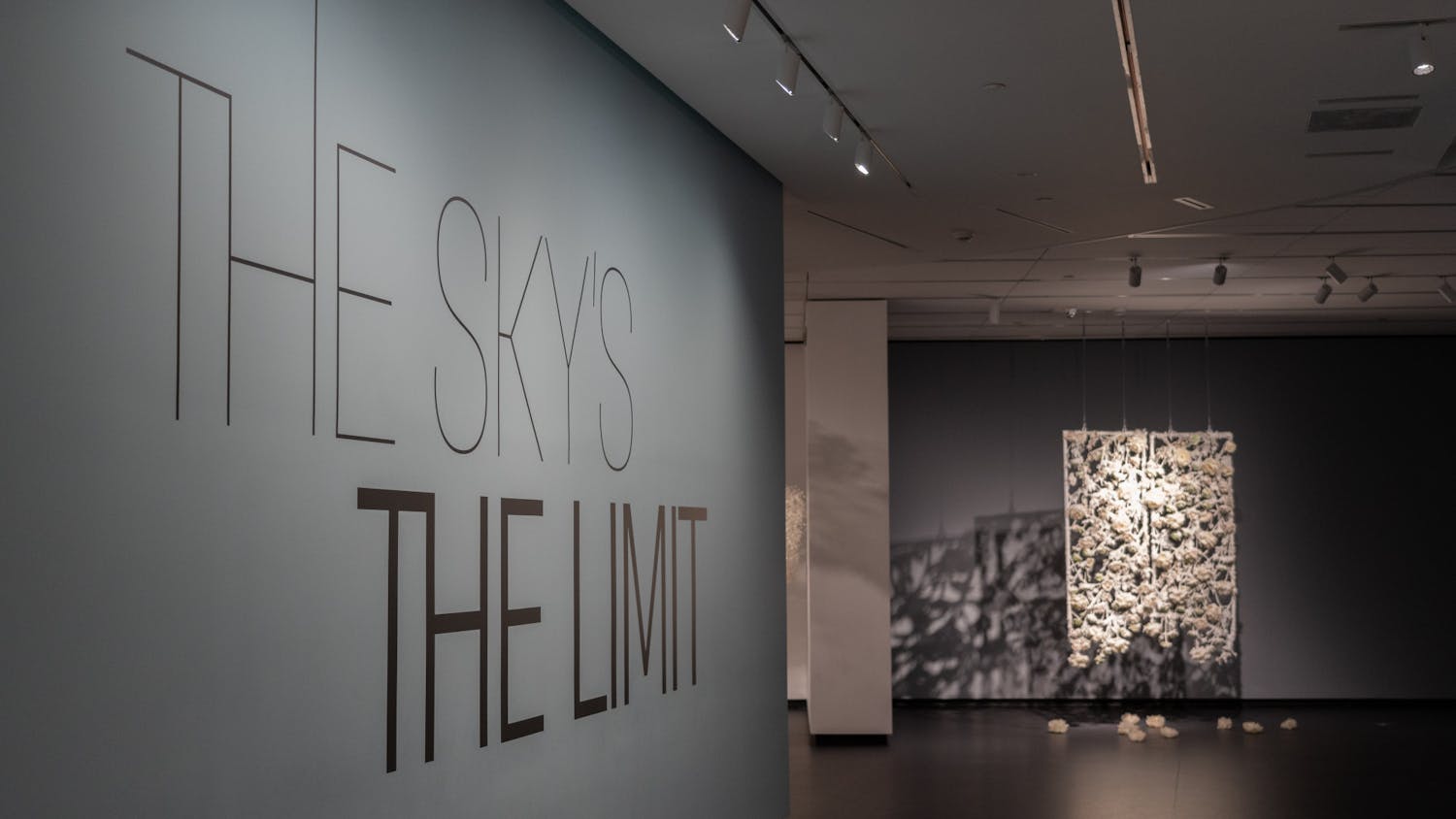The image is set inside a spacious museum room featuring various elements. On the left side of the image is a light gray wall with black text that reads, "The sky is the limit," where "the limit" is in bold lettering, while "the sky" is in thinner font, with the 'H' extending upward towards the ceiling. Adjacent to this wall is a white pillar, and just beyond it, there's an opening leading to another section of the museum. 

In the background against a gray-colored wall, there's an intriguing art installation hanging from the ceiling. This installation consists of two rectangular frames suspended by four wires, containing what appears to be plant branches or some kind of organic material, with some fragments scattered on the floor beneath it. The floor itself is a brown tone, possibly wood or tile. The installation casts multiple shadows due to the overhead spotlights. The ceiling of the room features track lighting and a vent, adding to the modern aesthetic of the space.